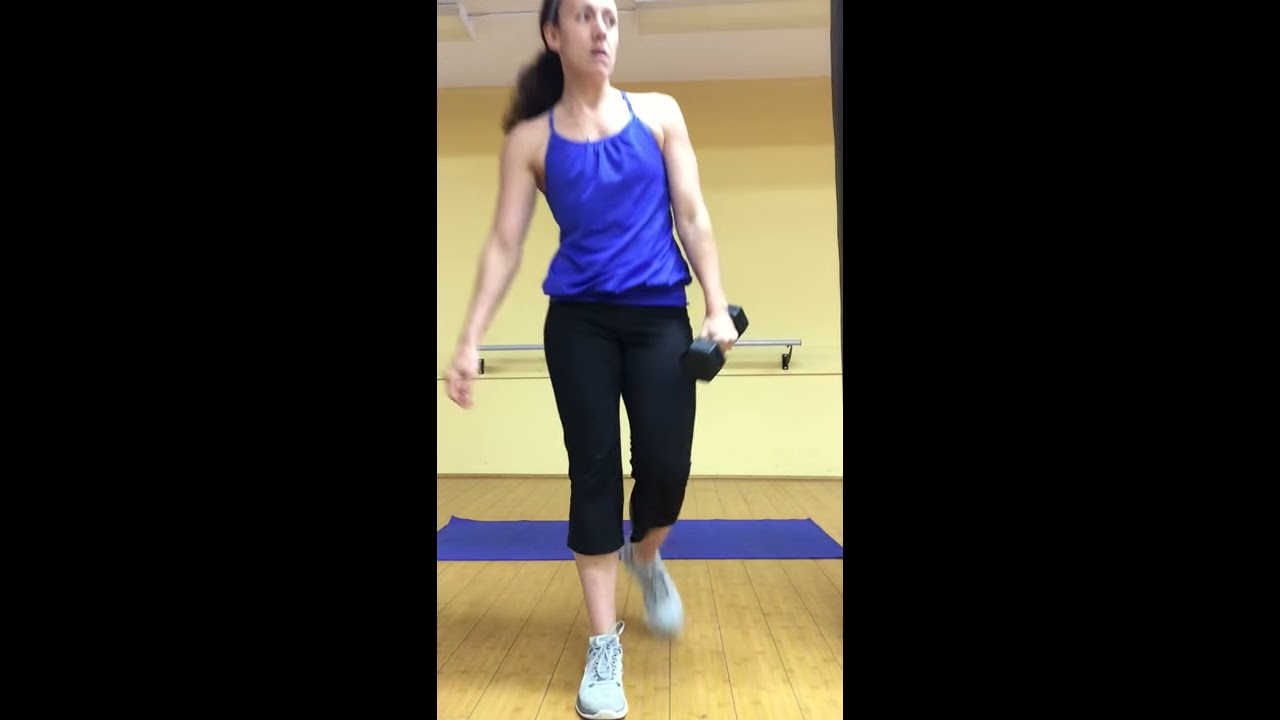The image captures a young woman, likely in her early 30s, engaging in a workout at a gym. Dressed in a blue tank top and black capri leggings, she also sports white tennis shoes and has her long, brown hair pulled back into a ponytail. She's holding a black dumbbell in her left hand while her right arm hangs loosely by her side. The scene is set on a wooden floor with individual slats visible, and a blue yoga mat is positioned behind her. The background features a light yellow wall with a fitness bar attached to it, and the ceiling is white. The image is somewhat blurry, indicating she's in mid-motion, possibly captured from a fitness video intended for social media platforms like TikTok or Instagram. The left and right thirds of the image are obscured by black rectangles, focusing attention on the central subject.